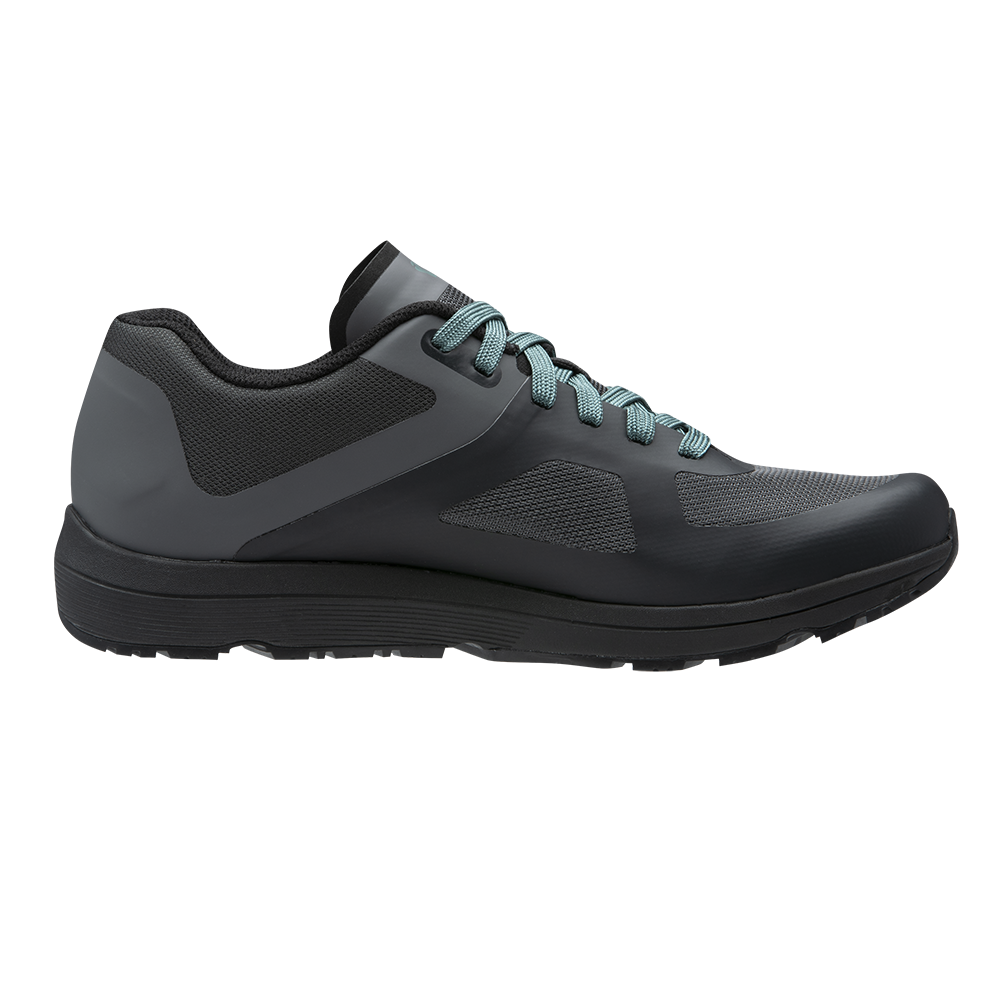This image features a detailed side view of a running tennis shoe against a stark white background, creating a clean, product-focused presentation. The shoe, likely designed for men, exhibits a color palette of black, dark gray, and light gray with striking teal blue laces that are fully laced up. The heel of the shoe is predominantly black, transitioning into a dark gray section that spans up toward the laces. This gray section includes a diagonal stripe from the lower heel to the top lace point. The shoe's upper part, particularly around the toe area, features light gray mesh for breathability, with an additional light gray mesh rectangle on the side. The tongue of the shoe is gray with black trim, peeking slightly above the laces. The sneaker has no visible branding, enhancing its sleek, modern aesthetic. The sole is made of black rubber with visible tread, indicating durability for running or athletic activities. The shoe appears new, with no visible wear, highlighting its pristine condition.